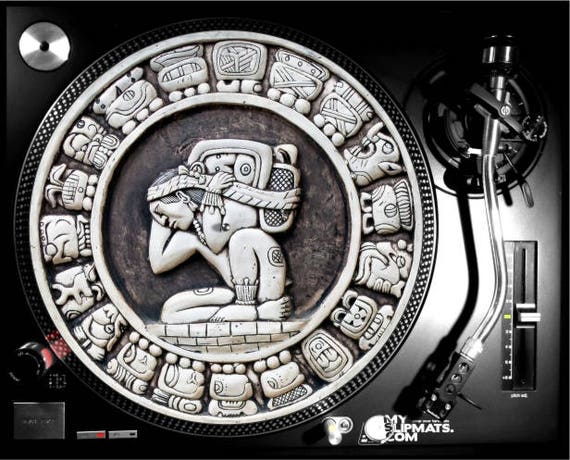The image depicts an intricate black-and-white composition, predominantly dark at the top. On the left, there's a large, silver-gray circle featuring a complex border adorned with carved designs. Inside the circle, a figure of a man is seen in a crouched position, his knee and foot on the ground, appearing to carry a heavy load on his back tied with a headband. The man, seemingly unclothed, has a pained expression with closed eyes, suggesting he is struggling under the weight he bears. Surrounding this central figure are various abstract shapes or tiny white figurines, forming a ring around him. The backdrop is a glossy black surface, resembling a record player, with a slightly curved, silver metal rod protruding on the right and adorned with some dark details. Additionally, a small shiny silver circle is discernible in the top-left corner of the black background.